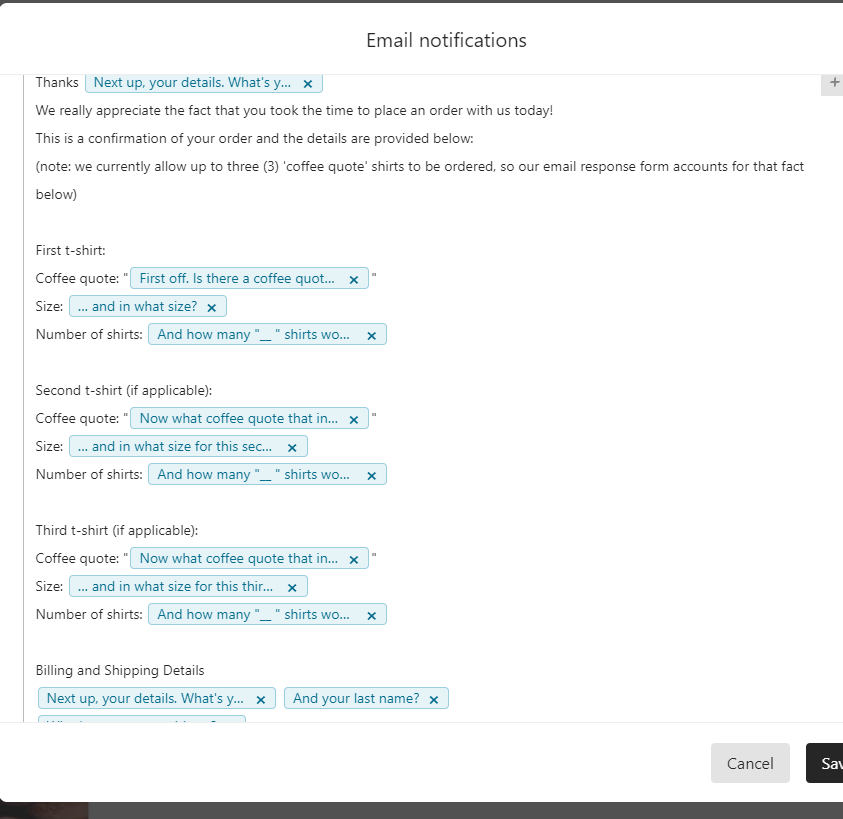**Email Notification Screenshot**

This screenshot captures the "Email Notifications" header displayed in black letters atop a white background. The main content is structured in several paragraphs, primarily in black text interspersed with blue buttons. The email appears to be an order confirmation, expressing gratitude for the recipient’s purchase and summarizing the order details.

The body of the email begins with a message of appreciation: “We really appreciate the fact that you took the time to place an order with us today.” The email confirms the order and provides specific details about the items ordered, noting that up to three coffee quote shirts can be purchased. This limitation is acknowledged in the subsequent email response format.

For each shirt ordered, the email lists the following details:

1. **First T-Shirt:**
   - **Coffee Quote:** Placeholder text indicating where the coffee quote for the first shirt would be.
   - **Size:** Placeholder for the size of the first shirt.
   - **Number of Shirts:** Placeholder for the quantity of the first shirt.

2. **Second T-Shirt (if applicable):**
   - **Coffee Quote:** Placeholder text for the coffee quote on the second shirt.
   - **Size:** Placeholder for the size of the second shirt.
   - **Number of Shirts:** Placeholder for the quantity of the second shirt.

3. **Third T-Shirt (if applicable):**
   - **Coffee Quote:** Placeholder text for the coffee quote on the third shirt.
   - **Size:** Placeholder for the size of the third shirt.
   - **Number of Shirts:** Placeholder for the quantity of the third shirt.

Throughout the email, placeholder text and ellipses indicate where further details or inputs are required. The option to exit the screen is also available, denoted by "X out." 

This email notification provides a structured yet interactive layout for customers to review their order details, make necessary adjustments, and confirm the specifics of each item ordered.